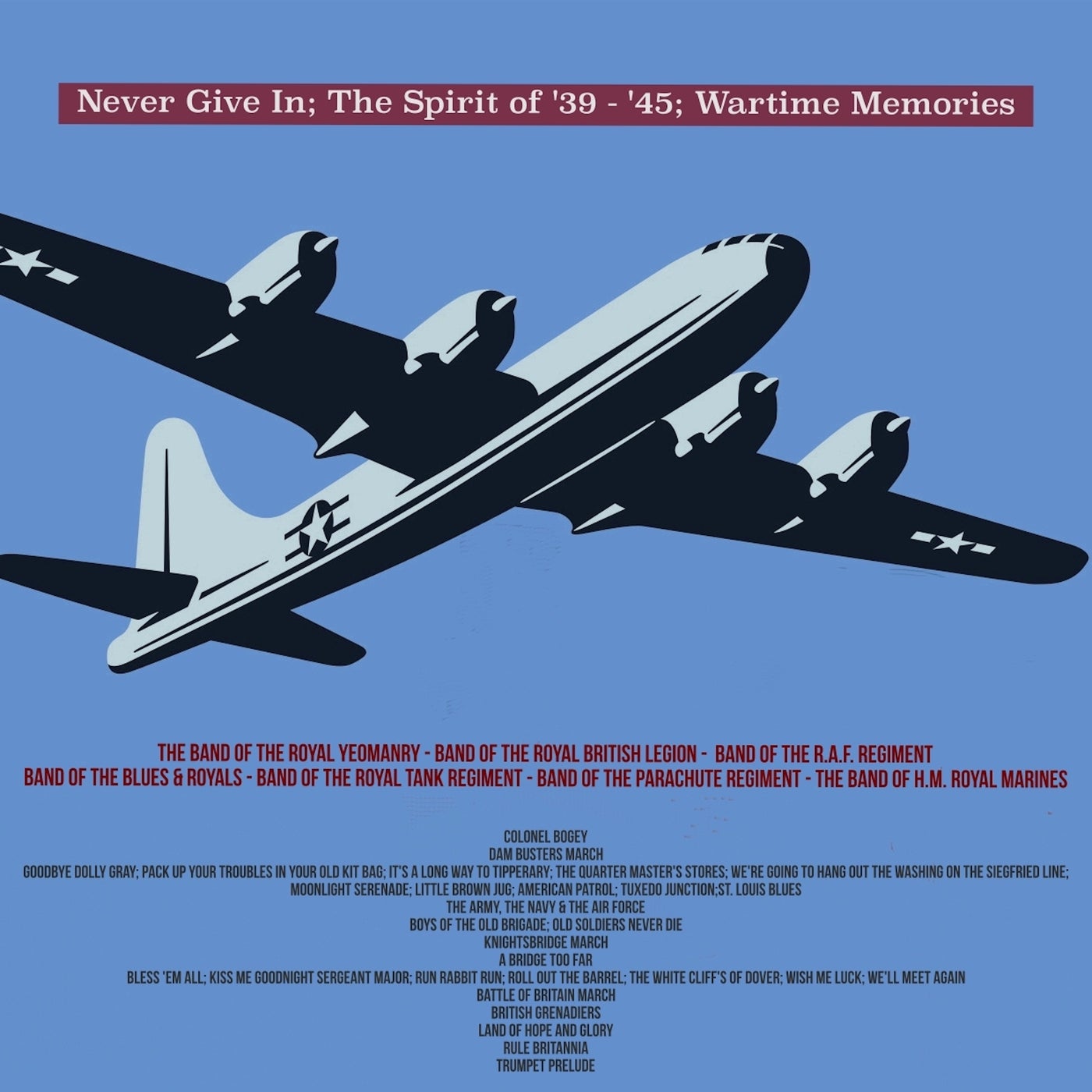This is an album cover featuring a military airplane in mid-flight, viewed from below. The light blue plane, accented with black shadows, dominates the center of the image against a solid blue background. The aircraft sports a distinctive five-point star logo in a circle with two horizontal lines on its side, and a similar star with minus signs on the wings.

At the top of the cover, white text set against a maroon banner reads: "Never Give In: The Spirit of '39 to '45 - Wartime Memories." Below the plane, maroon text lists the bands featured on the album: The Band of the Royal Yeomanry, Band of the Royal British Legion, Band of the RAF Regiment, Band of the Blues and Royals, Band of the Royal Tank Regiment, Band of the Parachute Regiment, and the Band of HM Royal Marines.

Centered beneath these details in black text are the numerous songs included in the album, such as: "Colonel Bogey," "Dambusters March," "Goodbye Dolly Gray," "Pack Up Your Troubles in Your Old Kit Bag," "It's a Long Way to Tipperary," "The Quartermaster's Stores," "We're Going to Hang Out the Washing on the Siegfried Line," "Moonlight Serenade," "Little Brown Jug," "American Patrol," "Tuxedo Junction," "St. Louis Blues," "The Army, The Navy, and The Air Force," "Boys of the Old Brigade," "Old Soldiers Never Die," "Knight's Bridge March," "A Bridge Too Far," "Bless Them All," "Kiss Me Goodnight, Sergeant Major," "Run Rabbit Run," "Roll Out the Barrel," "The White Cliffs of Dover," "Wish Me Luck," "We'll Meet Again," "Battle of Britain March," "British Grenadiers," "Land of Hope and Glory," "Rule Britannia," and "Trumpet Prelude."